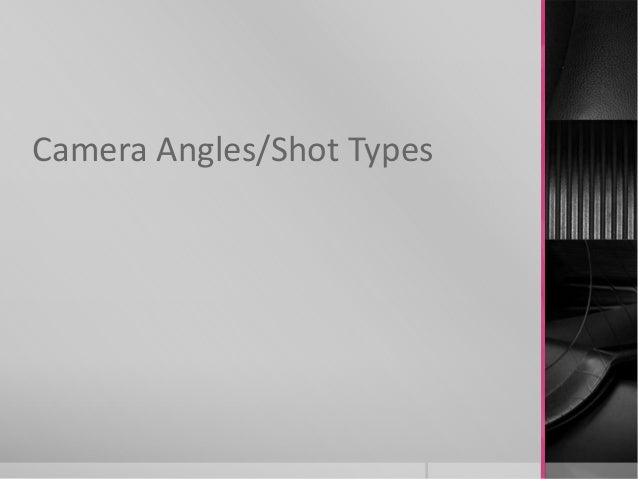The image is a rectangular, slide presentation with a solid medium gray background. About 85% of the image, on the left, is a light gray square, occupying most of the width. Around one-third down from the top of this gray square, there's large dark gray text that reads "CAMERA ANGLES / SHOT TYPES." This text spans roughly 70% of the horizontal space. On the right side of the image, a pink line runs vertically from top to bottom, adjacent to the gray square.

To the right of this pink line, taking up the remaining 15% of the image, are three vertically stacked areas. The top two areas are equal in height and feature gradients transitioning from black to lighter shades of gray, with the upper one being completely dark at the top and the bottom showing some indistinct shapes. The middle area features alternating grooves with varying shades of gray. The bottom area is the tallest and also very dark, showing shadows and a few highlights of a curved object, potentially a piece of metal. The entire bottom section of the image has a thin light gray band.

Together, this composition emphasizes how different camera angles and shot types influence the appearance of surfaces under various lighting conditions.